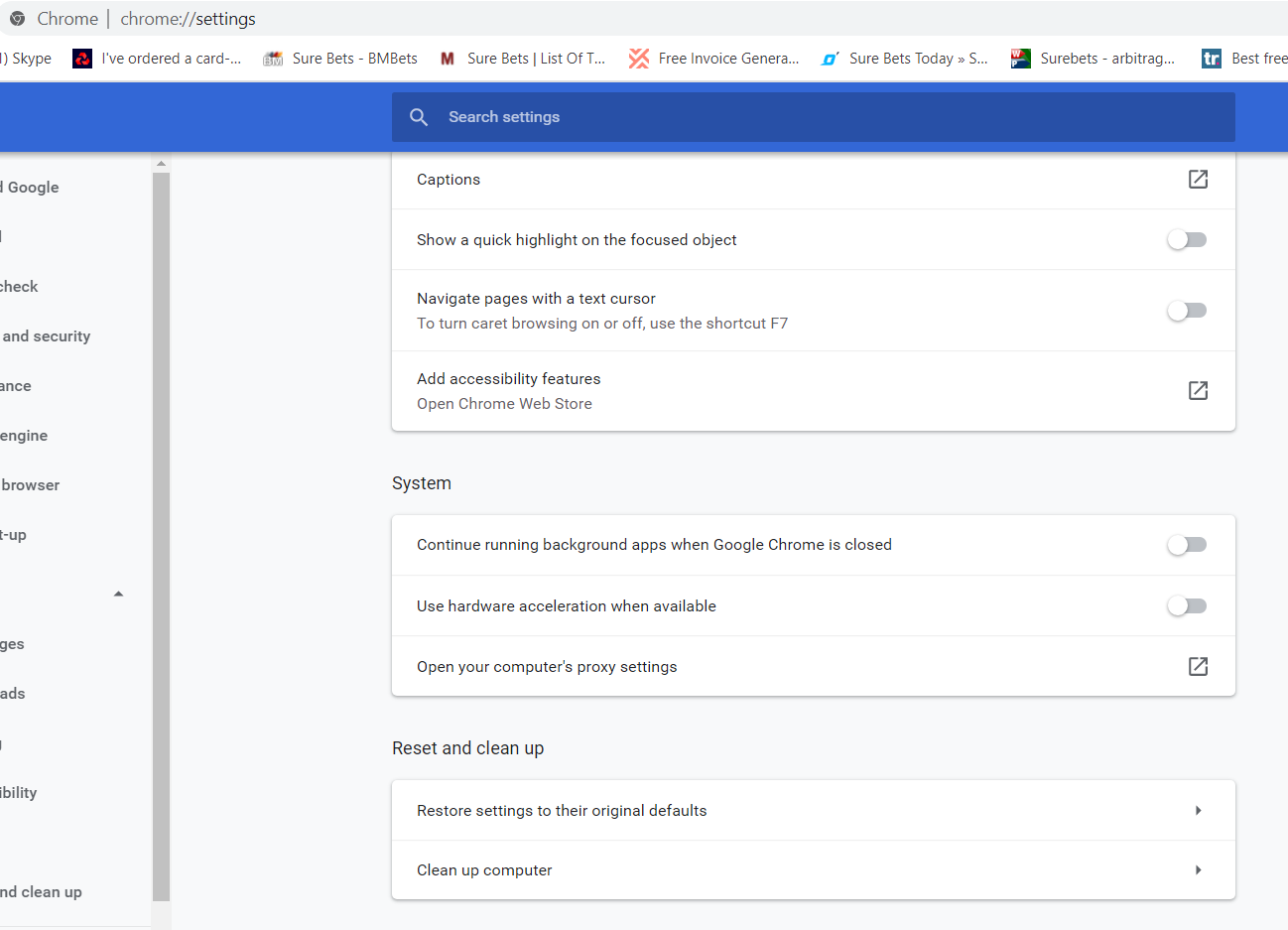This image is a screenshot of a desktop displaying the Google Chrome settings menu. At the top left corner, the URL "chrome://settings" is visible, indicating the current settings page. Just below this URL bar, there is a bookmarks bar containing several labeled bookmarks: "I've ordered a card," "SureBets," "SureBets," "Free Invoice Generator," "SureBets today," and "SureBets - Arbitrage." 

Further down, a horizontal blue bar spans the width of the page, featuring a prominent "Search settings" button. On the left side of the screen, there is a cropped vertical navigation bar, partially visible, which provides access to different settings categories.

The main section of the page is divided into three white boxes. The topmost box, titled “Accessibility,” includes the options: "Show a quick highlight on the focused object," "Navigate pages with a text cursor," and "Add accessibility features." Each option is accompanied by a corresponding icon to the right.

The middle box is labeled "System" and contains the settings: "Continue running background apps when Google Chrome is closed," "Use hardware acceleration when available," and "Open your computer's proxy settings."

The bottom box, under the heading "Reset and Cleanup," has two selectable options with right-facing arrows on their right side. These options are: "Restore settings to their original defaults," and "Clean up computer." 

The overall layout showcases a structured and user-friendly interface, aiding users in navigating and customizing their Chrome browser settings.